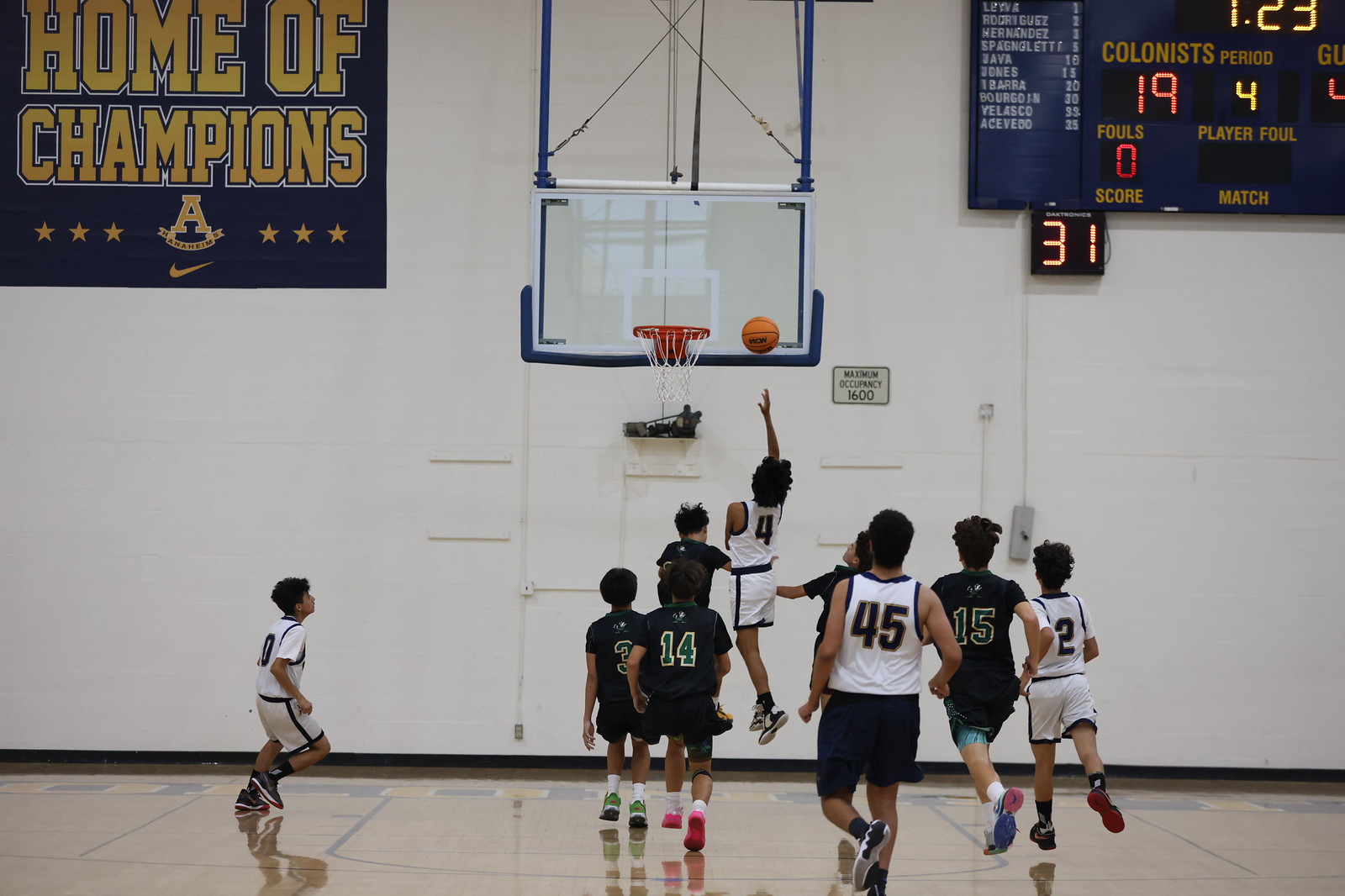The photograph captures a dynamic moment of a basketball game played by young boys, likely between the ages of middle school and early high school. It takes place in a gymnasium with white walls and a glossy, brown floor marked with black lines. The gym's ambiance is set with a poster in the upper left corner that reads "Home of Champions," and a scoreboard on the upper right showing a score of 19, with one team named Colonist and the other partially named GU. The basketball teams are distinguished by their uniforms; one team wears black and white tank tops with shorts, while the opposing team wears entirely black attire. The focal point of the image is a young player from the black and white team, captured mid-air as he shoots the ball towards the basket. The gymnasium's maximum occupancy is noted as 1600, with about eight players visible on the court, immersed in the heat of the game.